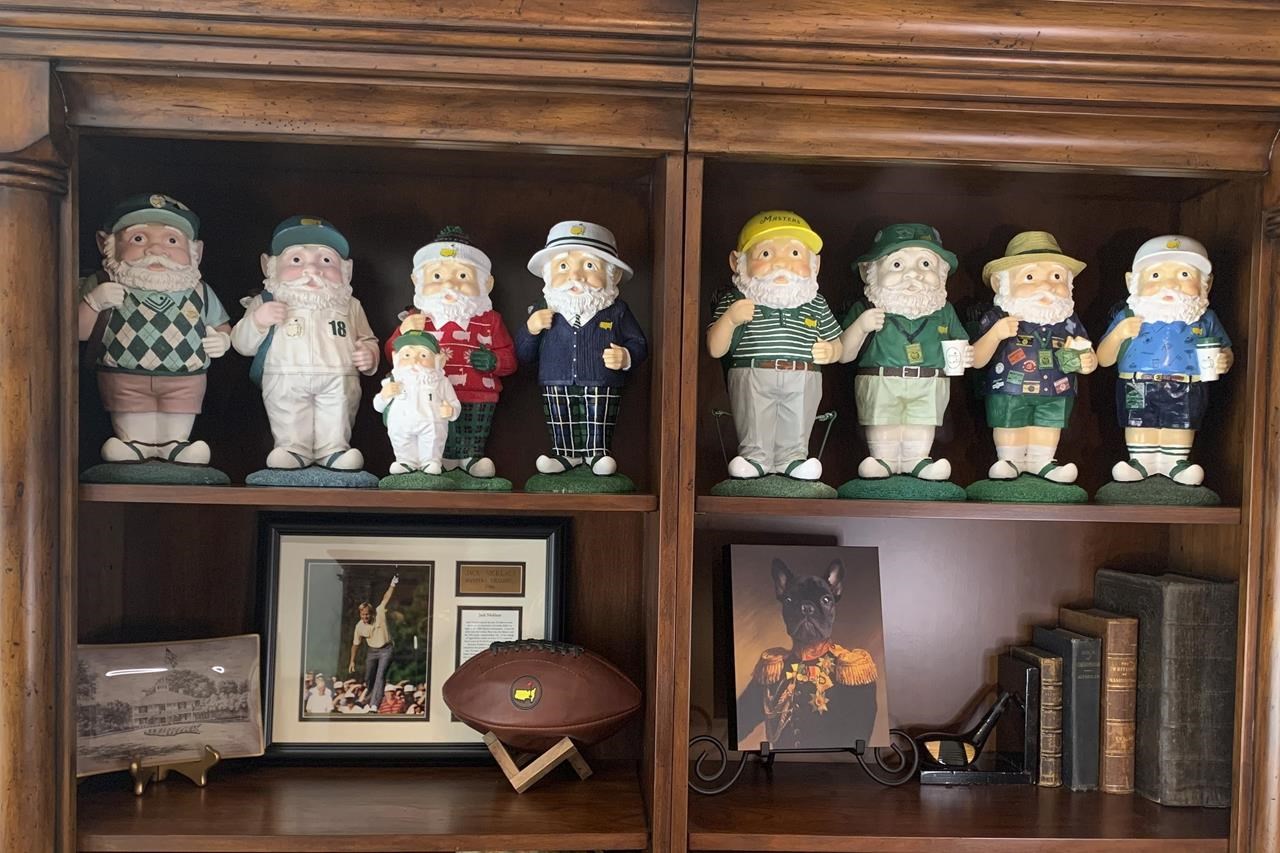This image features a highly polished, dark brown wooden cabinet with four rectangular shelves divided by a thin vertical slit, implying that two cabinets have been placed side by side. The top shelves are adorned with a collection of porcelain figurines, each depicting an old man in different costumes performing various activities. From left to right, the costumes include a golfer with checked sweaters and a bag of clubs, a man in sweats with the number 18, a man in a Christmas sweater, a sailor with a captain’s hat, a man in a striped shirt with a yellow hat, a hiker with a green fisherman's hat, a man in a shirt with stickers, and lastly, a man in a blue shirt and white hat holding a cup. 

On the bottom left shelf, there's a framed photograph of a house, a framed image of a man performing an athletic activity, and an award with a plaque. Additionally, a leather football rests on a wooden stand. The bottom right shelf displays an artistic print of a military officer with the head of a black dog, dressed in an ornate uniform with gold braids and epaulets. This shelf also contains a series of older-looking, dark-colored books held upright by a bookend featuring a golf club end.